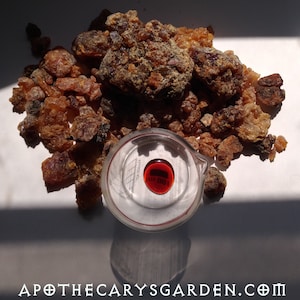The photograph from apothecariesgarden.com presents a detailed top-down view of an intriguing scene. A central circular case with a clear surface holds a polished, amber-colored round gemstone with a prominent red center, resembling a drop of red liquid. Surrounding this case is a scattered pile of rough gemstones, featuring a variety of rich hues including reds, amber, browns, and oranges. The rough stones exhibit intricate inclusions and brown matrix, reminiscent of crystalline structures or popcorn-like shapes. This setup is bathed in sunlight, just beyond a stark line of shade, creating a striking visual contrast. The background seems to transition from gray to white, possibly illuminated to create a soft flash of light. At the bottom of the image, the website "apothecariesgarden.com" is elegantly inscribed in white text.